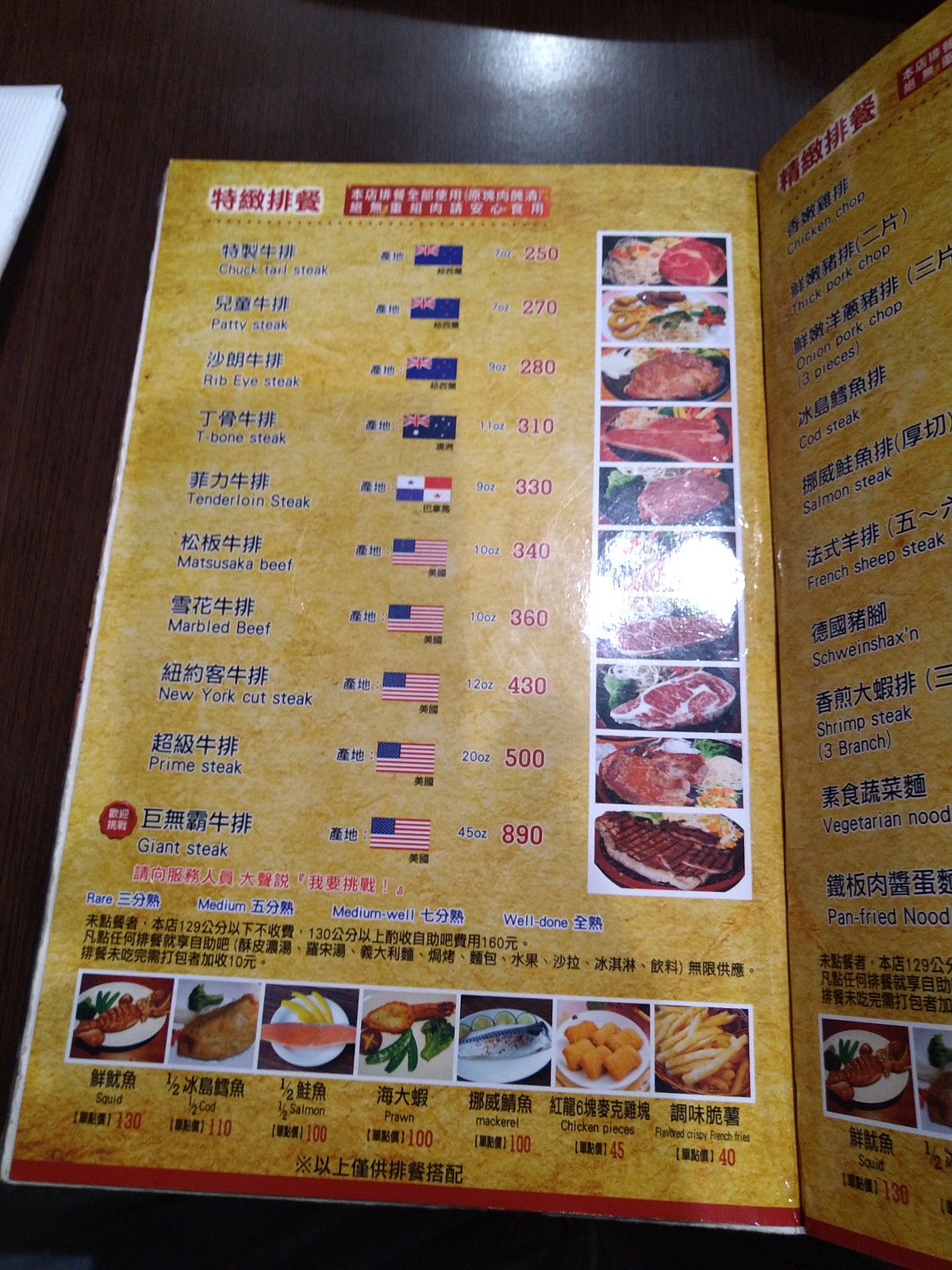The image showcases the inside of an Asian menu with a distinctive, textured background featuring lighter tan and darker brown mottled patterns. At the top center, there is a prominent red rectangle, and to its upper left, a white rectangle with kanji characters, indicating the menu's Asian origin. The menu is structured with a vertical row listing various meats, likely different cuts of steak, totaling ten options. The two steaks positioned in the center of the row are partially obscured due to the reflection of the camera flash.

On the far left, the dish names are displayed in kanji script with English translations directly below. Adjacent to this, a column of country flags culminates in a few American flags at the bottom. To the right of the flags are the prices for each dish, and next to these prices, high-quality images of the steaks are provided.

The bottom section of the menu features vivid photographs of side dishes, each accompanied by detailed descriptions in both kanji and English, ensuring clarity for both native and international diners.